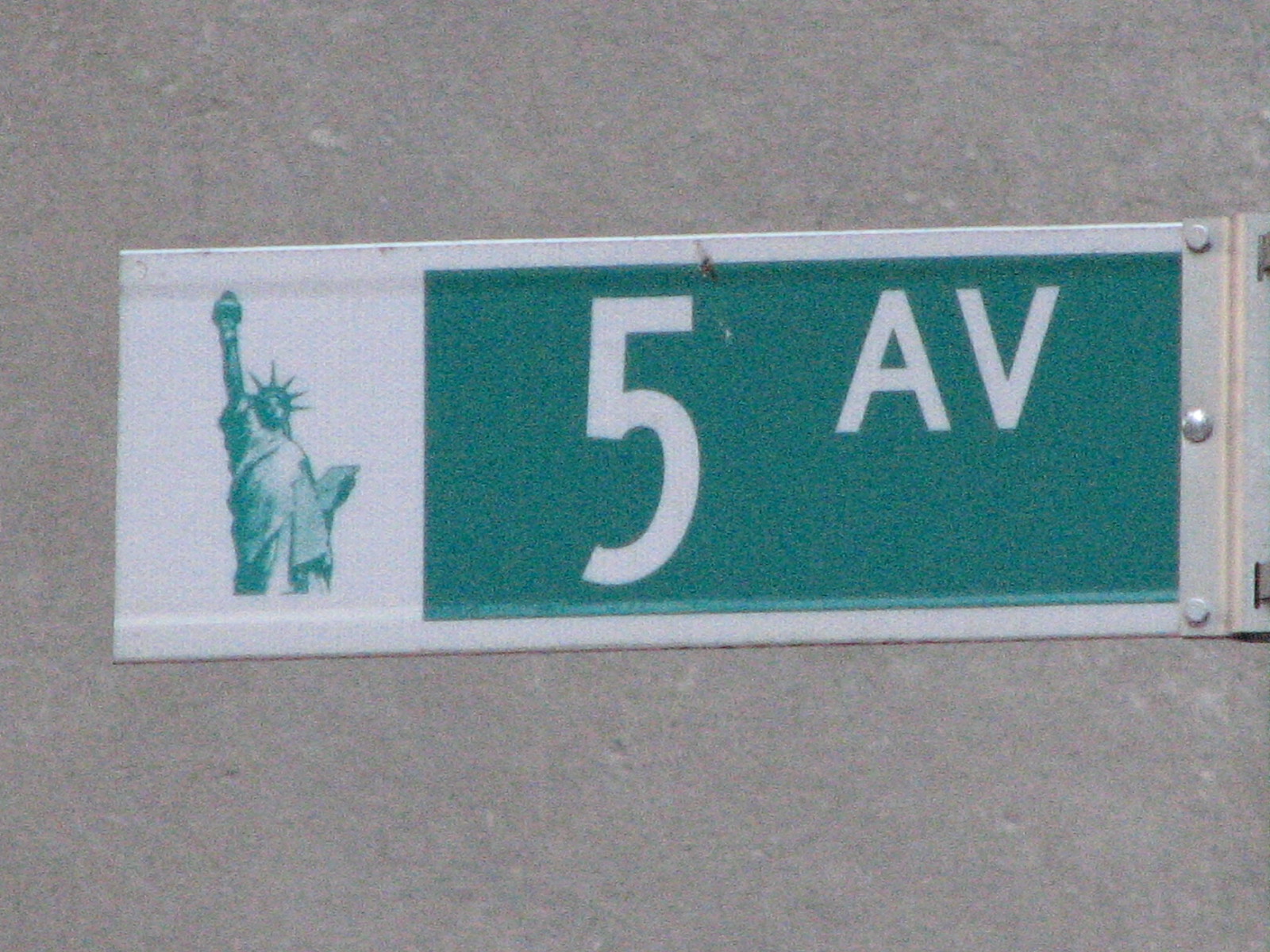The image features a textured background in light to medium gray with scattered white spots throughout, adding depth and contrast. At the center-left of the photo stands a prominent street sign with distinct elements. The sign itself is predominantly green with white lettering that reads "5AV." On the leftmost part of the sign, there is a white section displaying an image of the Statue of Liberty in green. The right side of the sign transitions into a light brown strip followed by three circular metallic fixtures. Further to the right, the sign shows a gray section with darker gray perforations arranged in a linear fashion, creating two small square holes through which the textured gray background is visible. The combination of these elements creates a complex and engaging visual narrative.